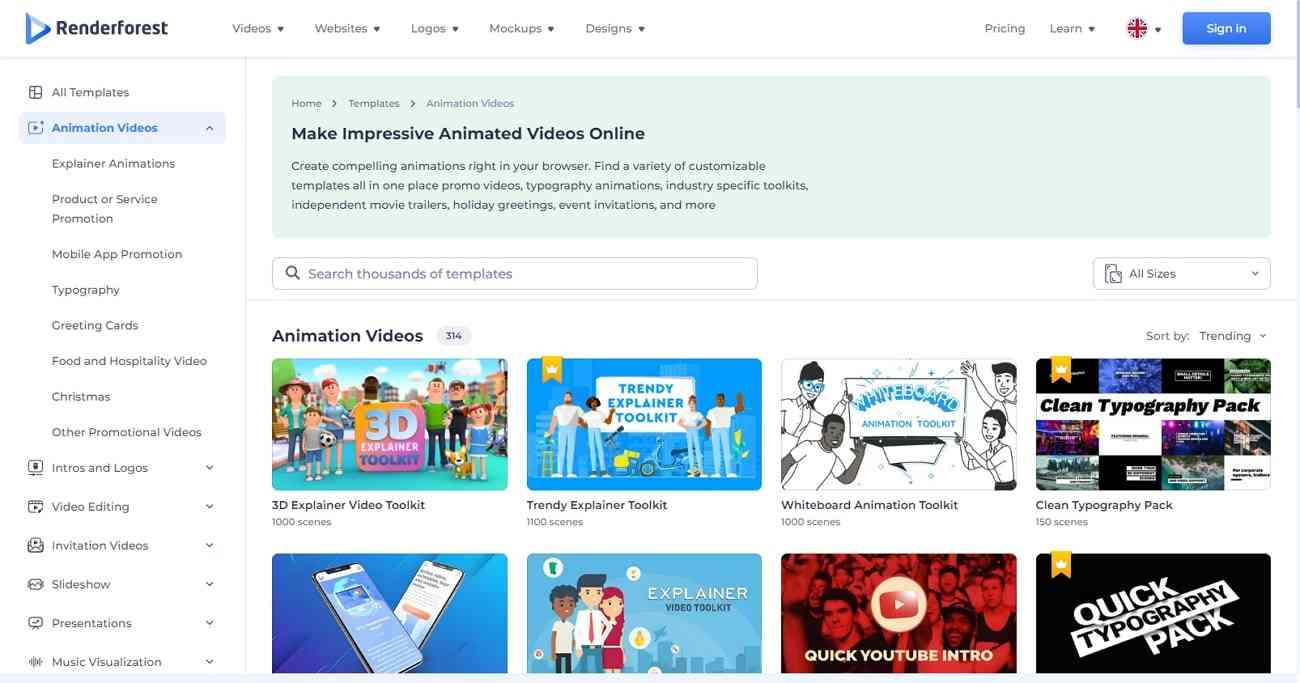In the top left corner of the image, there is an icon resembling a blue triangle tilted on its side, accompanied by the text "Render Forest." The categories listed include "Video," "Websites," "Logos," "Mockups," and "Designs." To the right of this section, the options "Pricing" and "Learn" are displayed, with the latter featuring a dropdown menu. Further to the right, there is a "Sign In" button. 

Below, the navigation menu includes options such as "Home," "Templates," and "Animation Videos," offering a variety of services and features. The content promotes the capabilities of creating impressive animated videos online, urging users to create compelling animations directly in their browser. It highlights the availability of a wide array of customizable templates, all conveniently accessible in one place. Specific template categories listed are "Promo Videos," "Typography Animation," "Industry-Specific Toolkits," "Independent Movie Trailers," "Holiday Greetings," and "Event Invitations," among others.

Underneath the search bar labeled "Search Thousands of Templates," are eight different thumbnail previews of various templates. The top left thumbnail is labeled "3D Explainer Video Toolkit," followed by another thumbnail labeled "Trendy Explainer Toolkit."